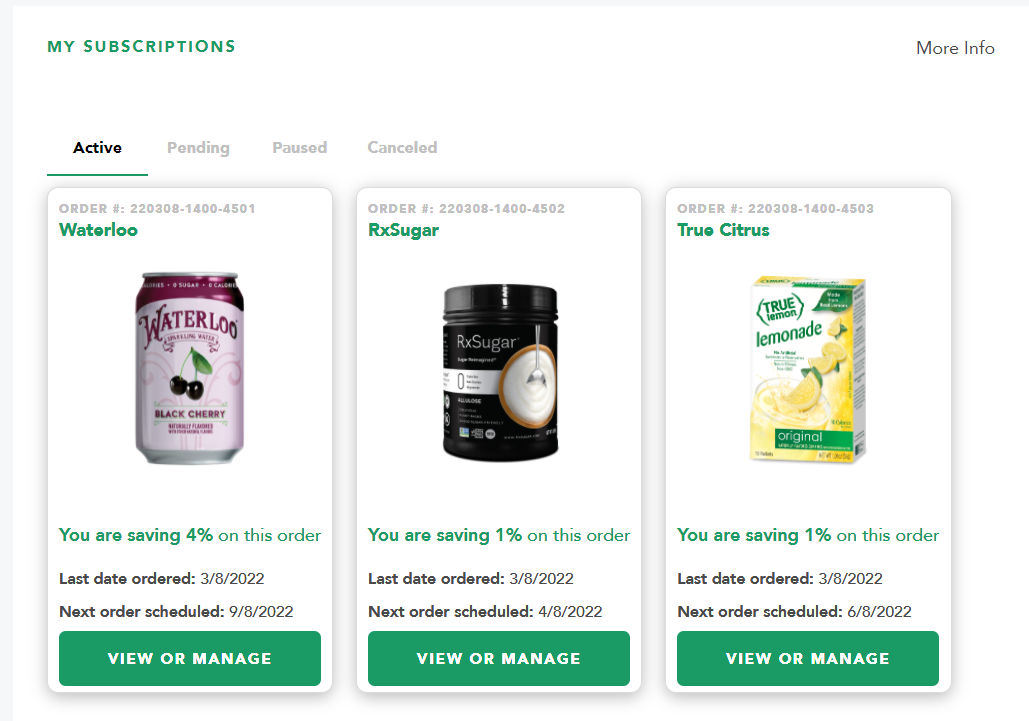A detailed screenshot depicting a user's subscription management page. At the top left, the heading "My Subscriptions" is displayed in green text against a white background. There are several tabs for navigating subscription statuses; the currently highlighted tab, labeled "Active," is in bold black text with a green underline. The adjacent tab labeled "Pending" is in gray, followed by two more tabs, "Paused" and "Canceled," also in gray.

Beneath the navigation tabs, three active subscriptions are listed:

1. **Waterloo Drink Subscription**: 
   - **Order Number**: [Displayed at the top]
   - **Brand Name**: Waterloo
   - **Product**: Black Cherry Waterloo
   - **Product Image**: A dark maroon red can of Black Cherry Waterloo
   - **Savings**: You are saving 4% on this order
   - **Last Order Date**: March 8, 2022
   - **Next Order Date**: September 8, 2022

2. **RX Sugar Subscription**:
   - **Order Number**: [Displayed at the top]
   - **Brand Name**: RX Sugar
   - **Savings**: You are saving 1% on this order
   - **Last Order Date**: March 8, 2022
   - **Next Order Date**: April 8, 2022

3. **True Citrus Lemonade Subscription**:
   - **Order Number**: [Displayed at the top]
   - **Brand Name**: True Citrus
   - **Product**: True Citrus Lemonade